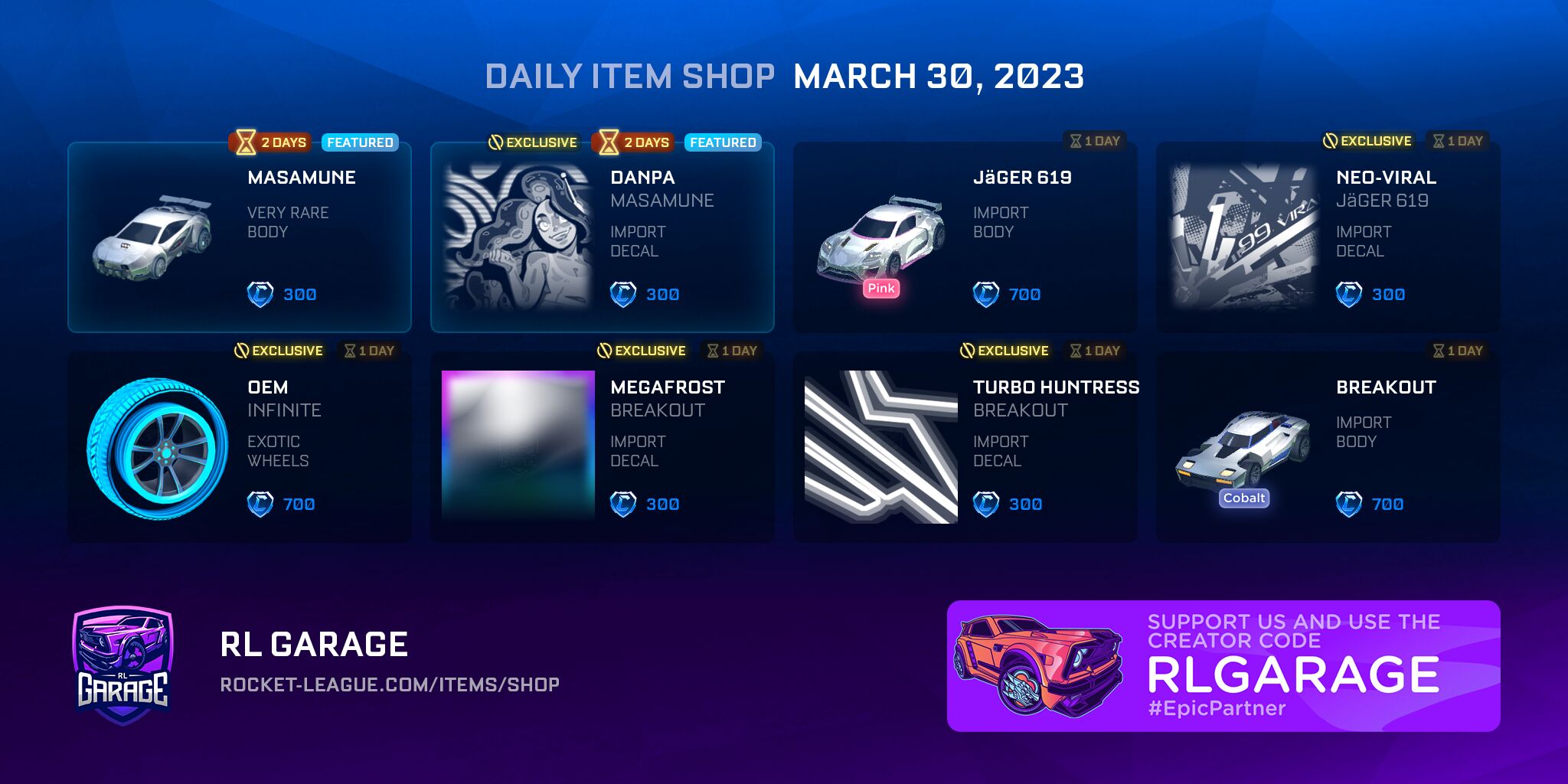A screenshot of the in-game shop in Rocket League, showcasing the daily item selection for March 30th, 2023. The shop features a two-tone gradient background, transitioning from blue at the top to purple at the bottom. 

In the bottom left corner, there is a purple badge labeled "Garage" in white text, adjacent to the letters "RL" and the words "Garage," representing Rocket League Garage. Below this, the URL "rocket-league.com/items/shop" is displayed. 

The bottom right corner features another badge, which reads "Support us and use the creator code RLGarage #EpicPartner." 

At the top center, there are two rows of items, each containing four distinct items available for purchase in the daily shop. The top row includes a car, a decal, an import body, and another decal, while the bottom row features exotic wheels, two more decals, and an additional import body.